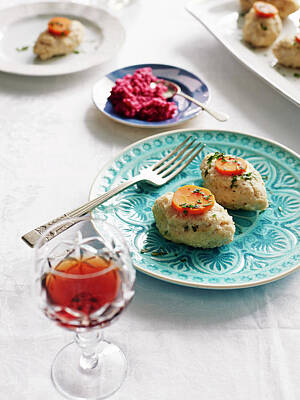Captured in the photograph is a detailed scene of a celebratory Jewish meal setting. The focal point is a turquoise plate featuring a decorative design, centrally placed in the image, which contains two oblong patties of gefilte fish, each adorned with a slice of bright orange carrot. To the left of the gefilte fish rests a fork, ready for service. Directly in front of the plate sits a glass goblet filled with red wine or possibly sherry, adding a touch of elegance and enhancing the festive ambiance. Surrounding this central plate are additional dishes - a nearby plate holds more gefilte fish, while a tray in the background is laden with similar fish patties, indicating a larger gathering. A chunky red sauce is also partially visible behind the main plate, adding a splash of vibrant color to the setting. This arrangement suggests a meal steeped in tradition, possibly tied to a Jewish celebration such as Hanukkah, with meticulously prepared dishes ready to be shared.